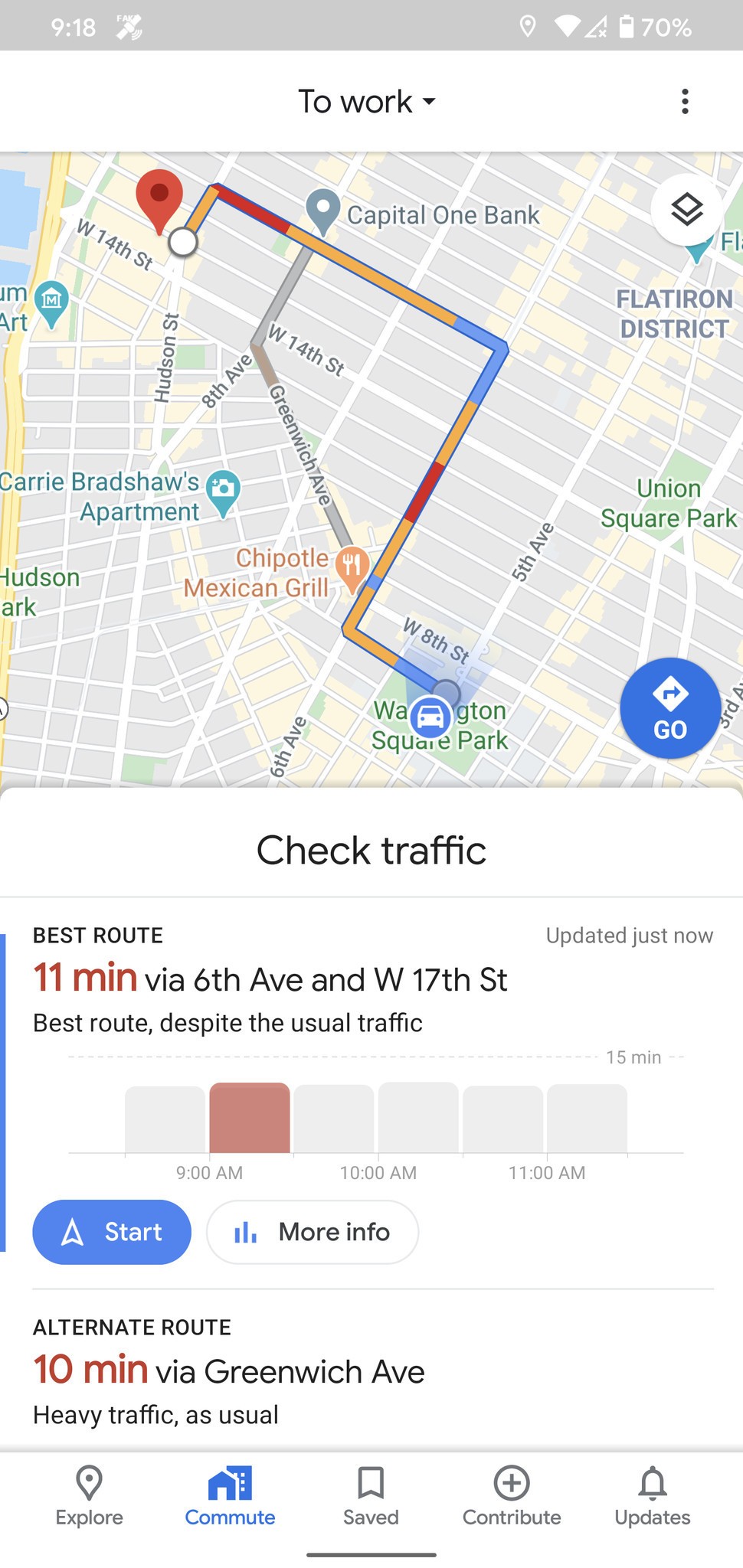**Description:** A screenshot captured from a smartphone displaying a Google Maps navigation interface. The top of the screen prominently features the text "To Work" in black. The main area contains a detailed map of New York City, recognizable by the labeled landmarks: Union Square Park on the right center and Washington Square Park at the bottom. A marker indicates "Carrie Bradshaw's apartment," further emphasizing the city's location.

The map highlights the best route from Washington Square Park to West 17th Street with a colorful line. Below the map, information about the route is provided: "Check Traffic: Best route 11 minutes via 6th Avenue and West 17th Street, best route despite the usual traffic," accompanied by a time indicator, "9:30," displayed inside a small brown square. 

Towards the bottom of the screen, options include a prominent blue "Start" button and a white "More Info" button. An alternate route is also suggested: "Alternate route 10 minutes via Greenwich Avenue, heavy traffic as usual."

At the very bottom, a navigation bar with icons for Explore, Commute, Saved, Contribute, and Updates is visible, providing quick access to additional features.